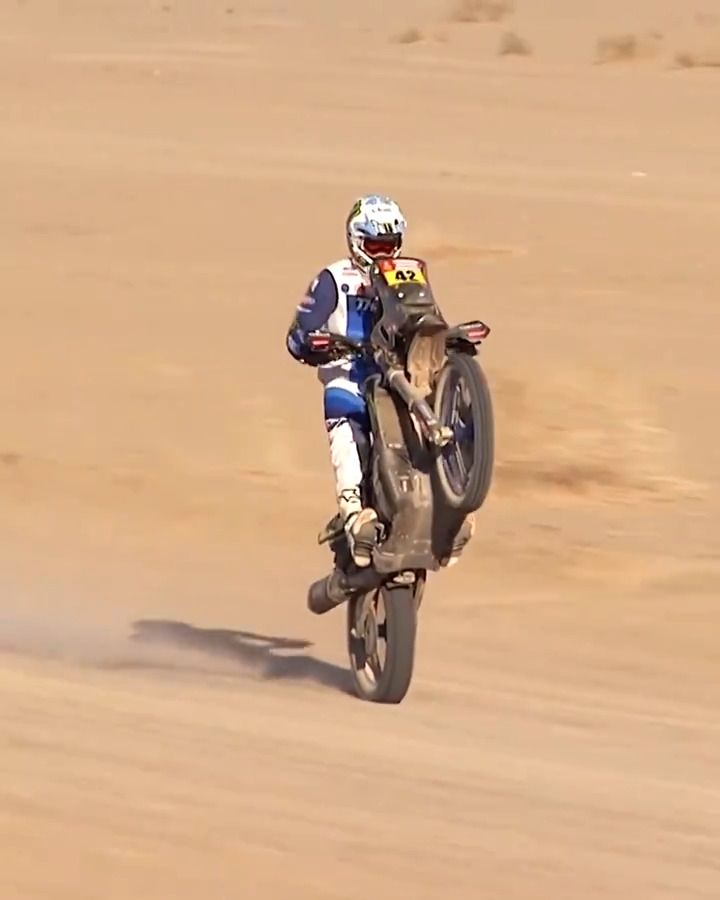The image is a realistic photograph captured by a photographer, featuring a captivating scene of off-road motorcycling in a desert setting. The image centers on a motorcyclist performing a dramatic wheelie, with the front wheel lifted off the sandy ground. The rider, clad in full protective gear, wears a white helmet with baby blue accents and an orange eye visor. Their outfit consists of long white pants featuring blue stripes above the knee, and a long-sleeved safety shirt with a navy blue square in the center and dark blue sleeves, likely adorned with sponsor patches.

The motorcycle, appearing slightly dusty and in sync with the sandy environment, is predominantly black and sports a distinct yellow number plate displaying the number 42 in bold black digits. The maneuver kicks up a visible trail of dust, accentuating the energetic and rugged nature of the scene. Surrounding the rider, the desert landscape is characterized by vast expanses of brown sand and sparse, dry green vegetation in the background. The photograph vividly captures the essence of off-road motorcycling against the stark, open backdrop of the desert, with no text intruding upon the image's raw and impactful visual storytelling.